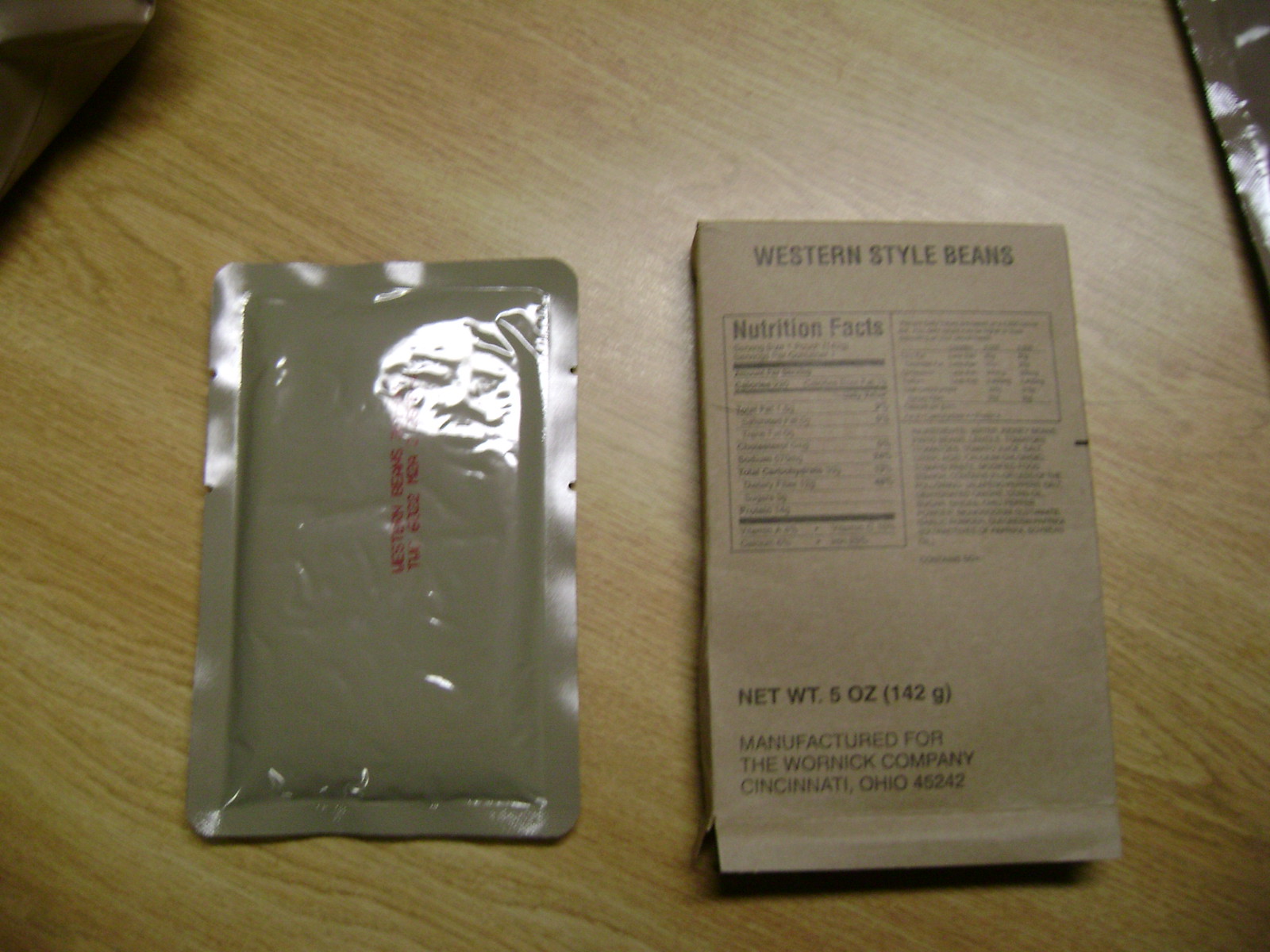This is a detailed indoor photograph featuring two components of an MRE (Meal Ready-to-Eat), typically issued to soldiers. Both packs are displayed on a pine-effect table. A noticeable dark shadow is present in the top left corner of the frame, while the edge of another MRE packet is slightly visible in the top right corner. The primary light source is an overhead light, which creates a reflective glare on the left-hand packet. 

The right-hand packet, made of brown paper, bears thorough printed information. At the top, it reads "Western Style Beans," followed by detailed nutrition facts. At the bottom, it specifies the weight and mentions the manufacturer: "Manufactured for The Warwick Company, Cincinnati, Ohio."

The left-hand packet, contrasting the right, is shiny and appears to be made from khaki green foil. Notably, it displays a manufacture date and an expiration date printed in red, providing vital information about its usability. The meticulous details captured in this photograph give a clear representation of typical MRE packaging as used by military personnel.